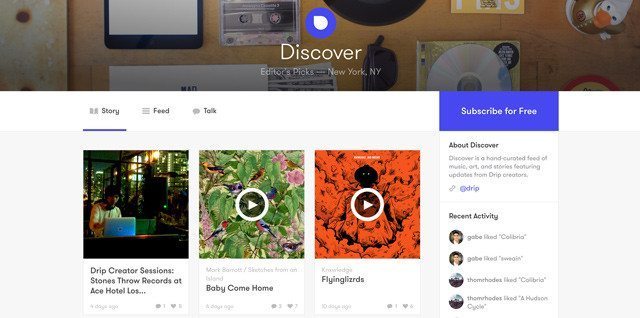This horizontal image, captured from a web page displayed on a computer or smartphone device, shows a detailed interface layout. At the top, a decorative background featuring various CDs and items hanging on a wall is partially visible. Overlaid on this background is the "Discover" icon accompanied by the text: "Discover," "Editor's Picks," and "New York, New York."

Beneath this, a white section of the interface presents icons for Story, Feed, and Talk. Below these, on a gray background, there are several icons and text listings. One icon displays a man at his computer, alongside labels reading "Trip Creator Sessions," "Stones Throw Records," "Ace Hotel," and an incomplete text starting with "Lost."

Following these listings are two video thumbnails with overlaying play buttons. The first video is titled "Baby, Come Home," and the second is "Flying Lizards."

To the right, a purple box with white text promotes a "Subscribe for Free" option. Below, a section titled "About Discover" contains a brief description of the Discover feature. Further down, a "Recent Activity" section shows a circular icon with a user's photo and highlights their recent interactions with the content.